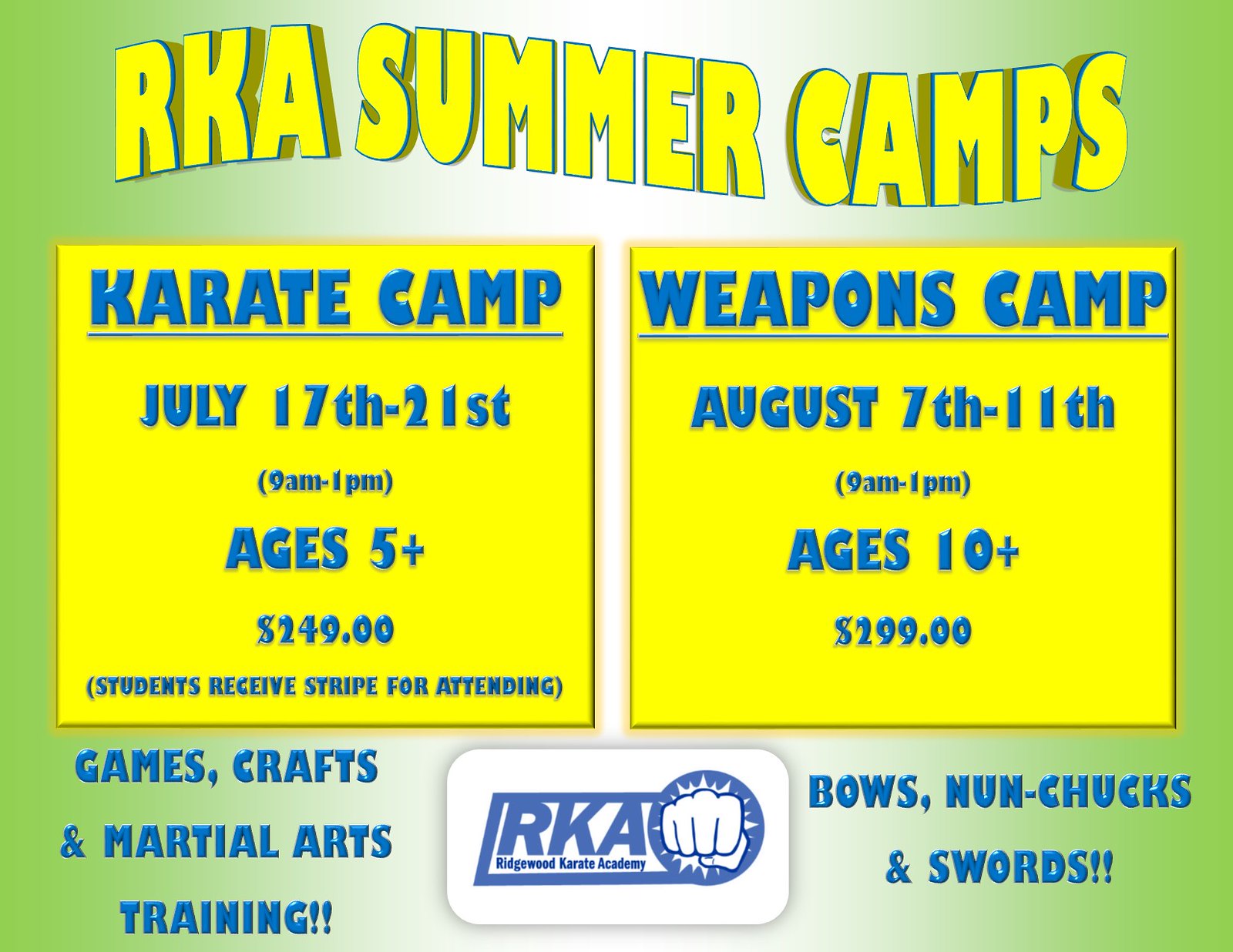This image is an online advertisement for RKA Summer Camps, designed with a green background that fades to white towards the center. At the top, the bold, shadowed title "RKA Summer Camps" stands out in yellow. Below, there are two yellow squares with blue text detailing the camps. On the left, the Karate Camp runs from July 17th to 21st, 9 a.m. to 1 p.m., for ages 5 and up, costing $249. Students attending this camp receive a stripe. On the right, the Weapons Camp is scheduled from August 7th to 11th, 9 a.m. to 1 p.m., for ages 10 and up, priced at $299. 

Below the camp details, the left section highlights activities such as "Games, Crafts, and Martial Arts Training," accented with exclamation points. In the center, the RKA logo features a fist bursting through a blue circle, representing Ridgewood Karate Academy. To the right, there's a focus on weapons used in the Weapons Camp, like bows, nunchucks, and swords, also punctuated with exclamation marks. This comprehensive poster encapsulates the essential information about the summer camps offered by Ridgewood Karate Academy.